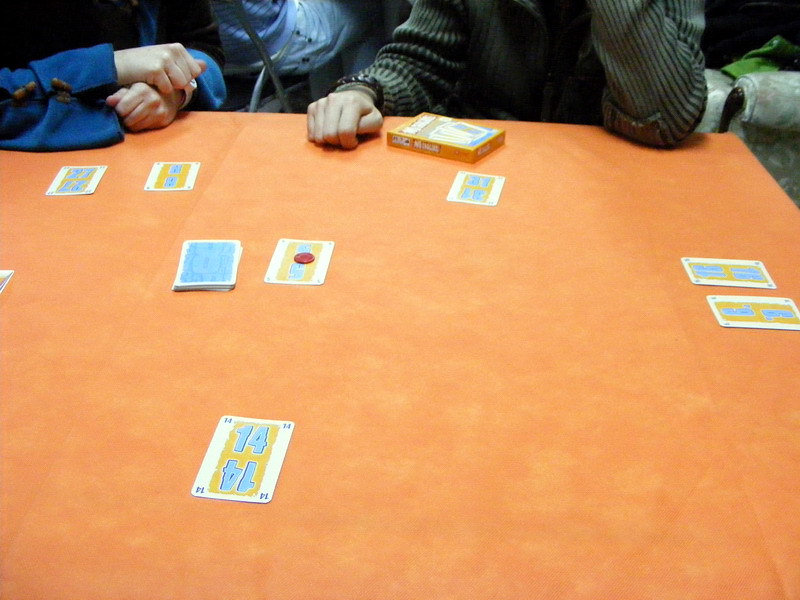A photograph captures a cozy indoor scene from a slightly elevated perspective, offering a detailed view of a lively card game in progress. In the upper right corner, a green, folded item is partially visible, adding a splash of color to the setting. Against this backdrop, a gray pot, which appears to have a crack, subtly hints at the environment's casual and homely nature.

In the background, a person dressed in blue is seated on a chair, observing the game. In the foreground, two individuals are deeply engaged in the card game. The player on the left sports a long blue jacket with brown ties along the sides and has their hands neatly crossed. The player on the right wears a gray sweater with long sleeves and an orange jacket, focusing intently on the cards spread out before them. Their game setup includes cards displaying various numbers and a red chip placed strategically next to the draw pile.

The game unfolds on a vibrant orange table, marbled with yellowish blotches that evoke a stunning, sunset-like hue. The table's surface features slight creases that add texture to the scene. Scattered cards around the table suggest that additional players, likely five in total, are involved in this engaging card game, even if they are not all captured within the frame. This detailed composition invites viewers to appreciate the nuances of this intimate and spirited gathering.